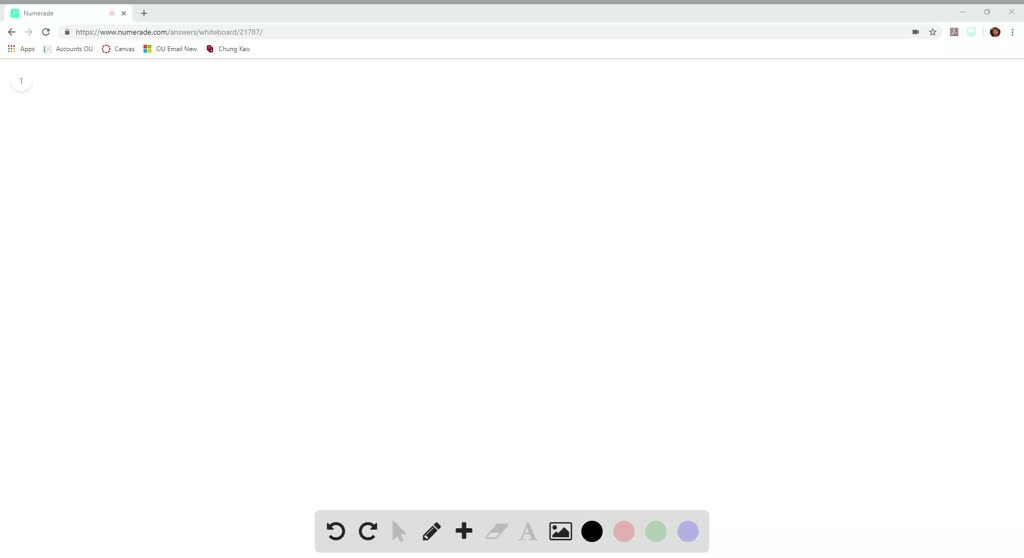This image depicts the interface of an online drawing tool that resembles Microsoft Paint but is presented within a web browser format. At the top of the page, there is a standard browser navigation bar. A white active tab is located on the left-hand side with a tiny green box adjacent to it bearing unreadable black text. This tab features a black "X" on the right for closing. Adjacent is a gray bar extending across the page, containing a black plus symbol. On the far right of this bar, typical browser icons appear: a minus sign for minimizing, a box outline for maximizing, and a black "X" for closing the window.

Below the browser navigation bar, on the left-hand side, are backward and forward navigation arrows, followed by a circular arrow icon for refreshing the page. A search bar is present next, though the text inside is illegible. Below this, a sidebar houses various icons: a multicolored "apps" logo resembling a rainbow, an unreadable black text icon, a red circle with white text, another icon with four quadrants of red, green, blue, and yellow colors, highlighting app availability.

The main workspace is a large, open area designated for drawing. Centered beneath this canvas is a gray toolbar featuring several icons: an undo arrow curving to the left, a redo arrow curving to the right, an upwards and leftwards pointing arrow, a black pencil symbol, a black plus sign, a gray eraser icon, a gray capital "A" for text, and a gray box with an image icon of a mountain and a sun in the upper left corner. Also present are four color selection circles in black, pink, green, and purple. This detailed interface serves as the platform's control center for creating and editing digital art.